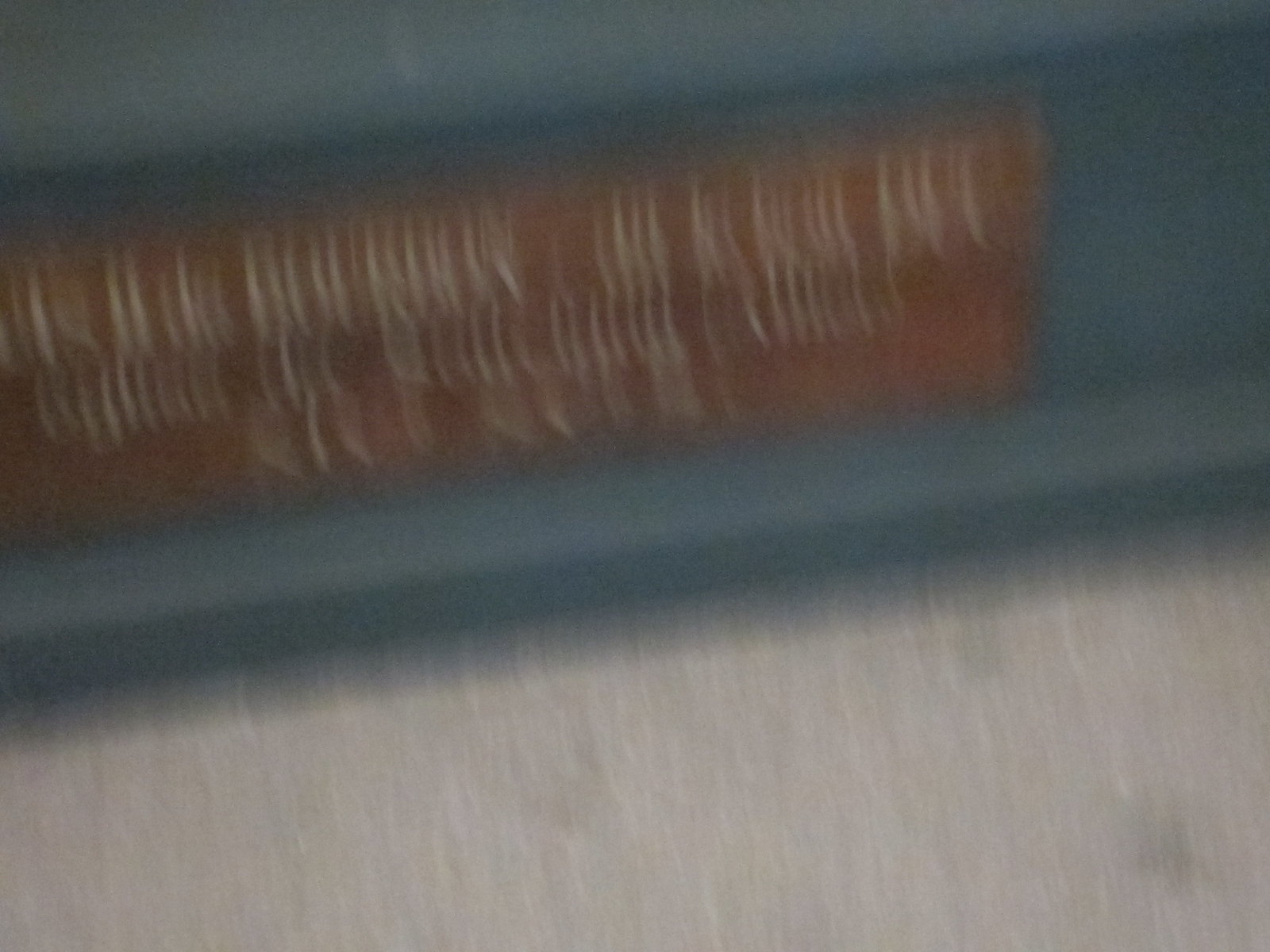This image is quite blurry and features a sign that resembles a brown banner affixed to an uncertain surface. The ground in the foreground appears to be a darker gray, possibly stone or asphalt, though its exact material is indiscernible. Adjacent to the sign, there is a small, dark-colored structure, possibly bluish, which seems like a low wall or partition one would find along the edge of a roadway with a curb beneath it. The sign itself has white lettering, but the text is unreadable due to the blurry quality of the image. The overall scene suggests an outdoor urban or semi-urban area.